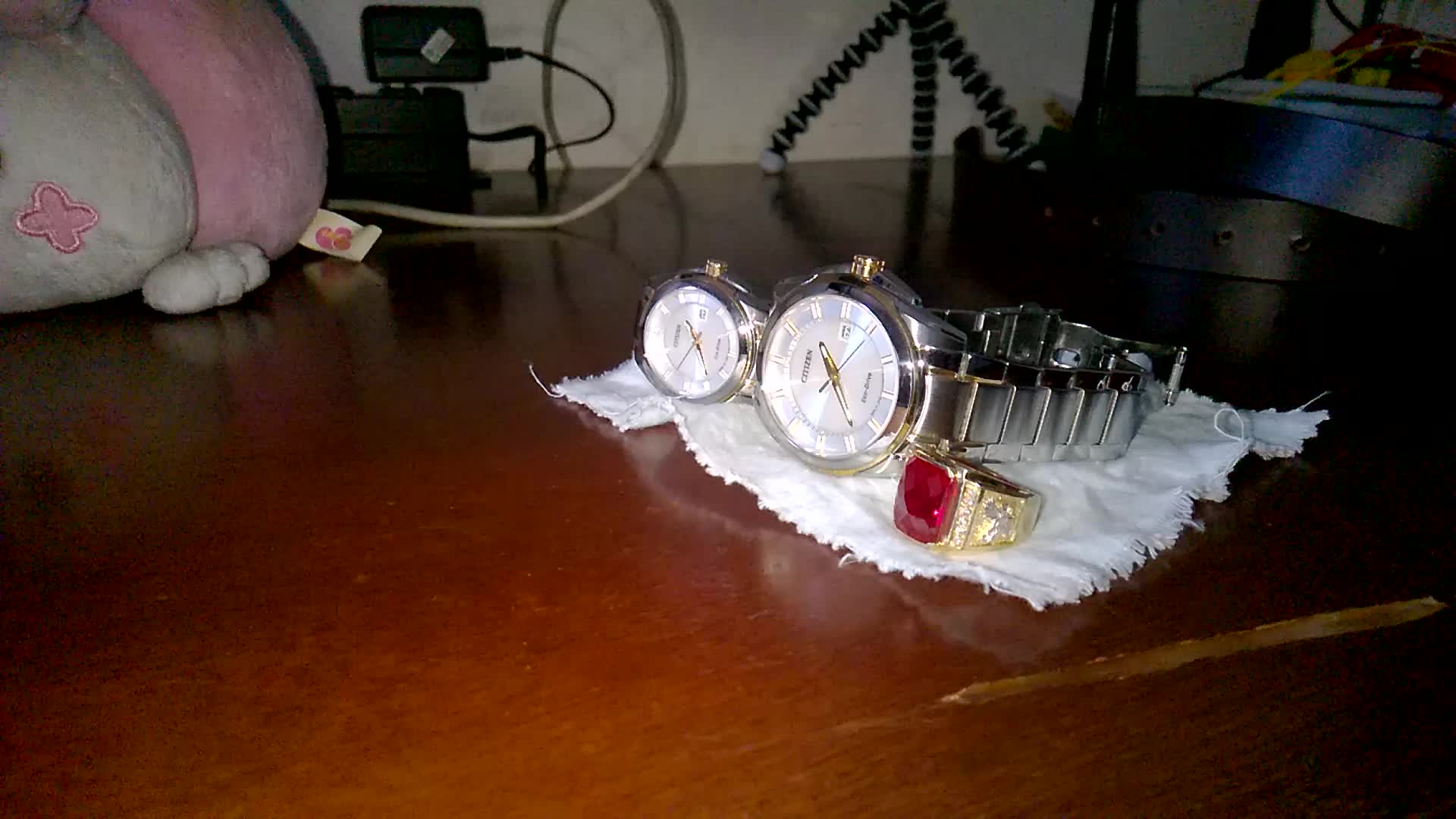This photograph captures a beautifully detailed arrangement on a wooden dresser top, featuring a pair of elegant his and her watches accompanied by a striking gold ring with a ruby. The dresser, made of brown wood, features a distinctive gouge on the right-hand side. Resting on a small, ragged-edged white cloth are the two silver-banded watches, each boasting a pearly white face with a touch of gold. The larger watch, intended for men, displays the time as approximately 2:38, while the smaller, matching watch intended for women is positioned slightly further back. Beside the watches, the thick gold ring, adorned with a square red stone, adds a luxurious touch to the scene. In the background, a pink and white stuffed animal with a distinguishing letter "T" can be seen, alongside some black belts, a black adapter plugged into a power strip, and the legs of a versatile tripod. The photograph, likely taken with flash, brings out the details of this intimate snapshot of personal accessories and everyday items.